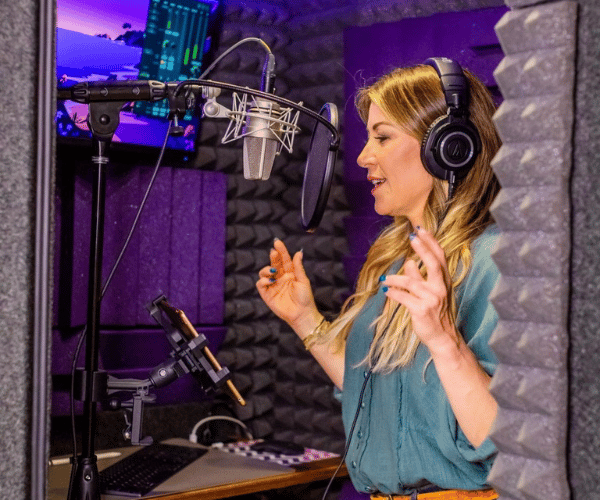In this detailed image, we see a Caucasian woman, likely in her late 30s or early 40s, engaged in a professional recording session inside a recording studio booth. The photo was taken from outside the booth. The woman has medium, shoulder-length dirty blonde hair with highlights, styled in loose waves. She is wearing black Audio-Technica headphones and a blue-green blouse with the sleeves rolled up to her elbows. Her bright blue fingernails stand out as she holds her hands up, bent at the elbows, keeping time or expressing herself.

The woman appears to be in the middle of singing or speaking, her mouth open as she faces slightly to the left. A professional microphone with a windscreen hangs in front of her, attached to a stand that features a holder for a tablet, from which she seems to be reading. The studio booth is equipped with grey and purple soundproofing materials, and there is a large disc-shaped recording screen situated near the woman's mouth.

In the background, various pieces of recording equipment are visible, including an LED monitor displaying levels and details with a purplish background, another screen showing a sunset wallpaper, a keyboard, and a mouse. The walls are adorned with black and grey sound-dampening materials, emphasizing the professional nature of the setting. This comprehensive setup, along with the visible excitement and focus of the woman, highlights the seriousness and professionalism of her recording session.